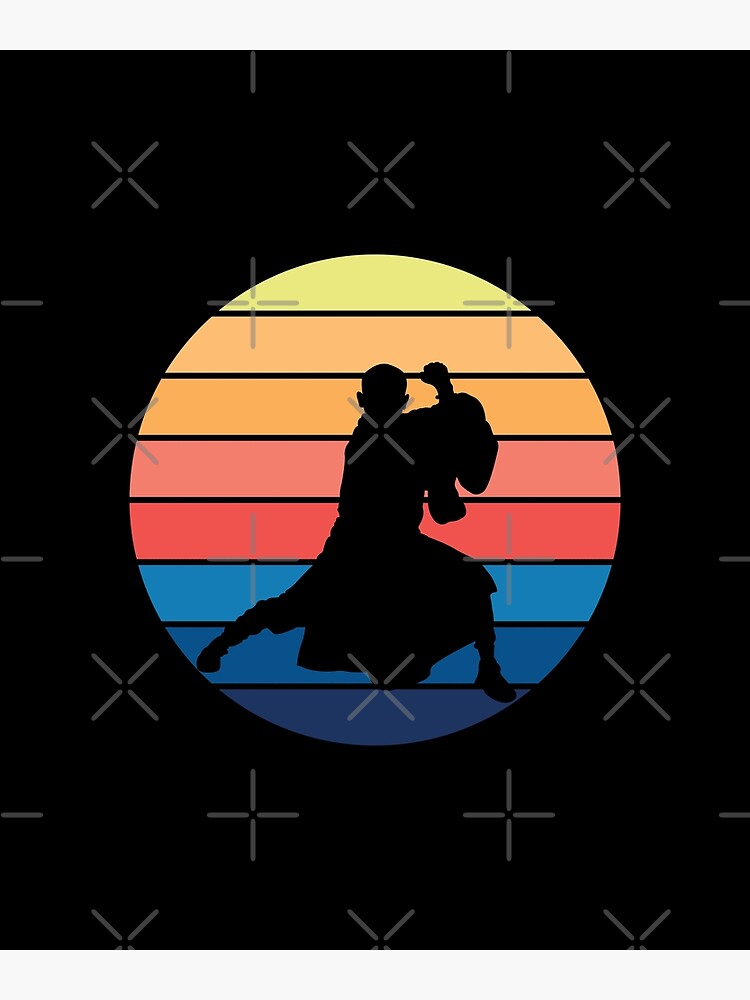The image in portrait orientation features a black background adorned with intricate gray patterns of alternating X's and plus signs. Central to the composition is a prominent circle, segmented into eight horizontal stripes of varying muted colors. From top to bottom, these stripes are pale yellow, peach, an orange-tinted peach, pinkish red, darker red, bright blue, a darker blue, and navy. 

Dividing each stripe are thin black lines that add to the layered effect of the image. Within this circle stands a black silhouette of a person in a dynamic pose, reminiscent of kung fu or a martial arts stance. The figure, possibly intended to evoke the image of a Jedi, faces forward with both ears visible, right arm bent at the elbow, and fist held near their head. Their legs are spread wide, with the right leg extended straight behind and the left leg bent forward as if in a lunge. The figure suggests motion and readiness, adding an almost combative energy to the otherwise static, colorful image.